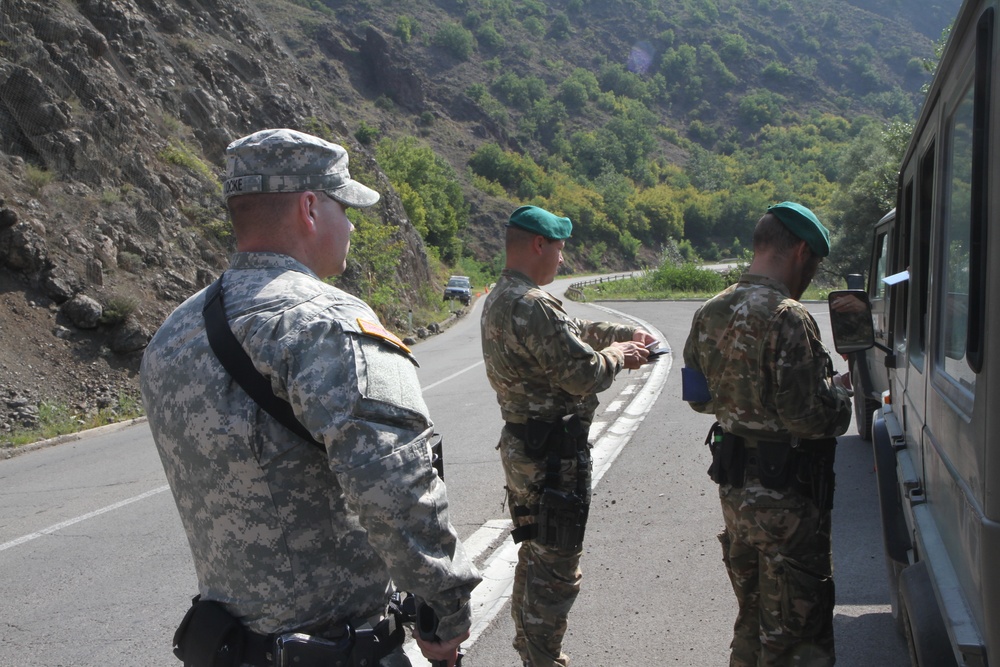In this detailed image, three soldiers in full camouflage fatigues and various military accessories are stationed on a winding mountain road. The two soldiers in the foreground, one wearing a matching cap and the other two donning green berets, are holding clipboards and appear to be taking down information. They are closely inspecting a large military vehicle parked nearby, which is partially visible in the lower corner of the photo. Behind them stands a third soldier in a different shade of uniform, suggesting he might be from a different branch or rank. The scene also features a second vehicle positioned ahead, with no occupants visible. The background is adorned with a mix of rocks, trees, and shrubs clinging to the mountainside, indicating the rugged and twisty nature of the road. The soldiers' focused posture and the presence of multiple vehicles suggest they might be conducting a routine checkpoint or inspection.